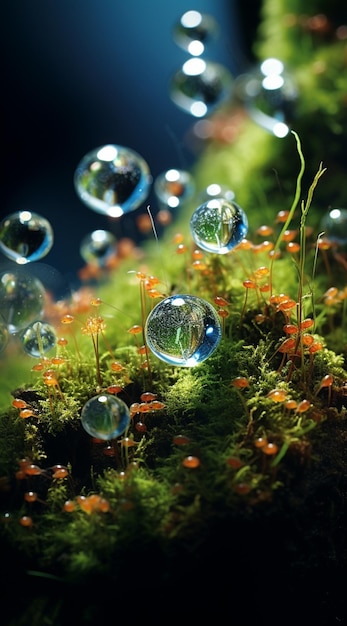This is a dark, landscape-oriented digital image that evokes an underwater or aquarium-like environment. The focal point is a variety of green, mossy underwater vegetation dotted with small orange or red egg-like pods or seeds. These vibrant elements stand out against a predominantly shadowy backdrop of deep blues and near-blacks. The lower half of the image is sharply in focus, revealing the intricate details of the plant life, while the background remains pleasingly blurred, contributing to the overall moody atmosphere. Large, reflective bubbles float amidst the scene, catching and scattering light, which adds a high-shine effect and a surreal, almost frozen or snow globe-like quality to the composition. The bubbles may be interpreted as water droplets or glass-like spheres, enhancing the enchanting and somewhat dystopian feel of the image.